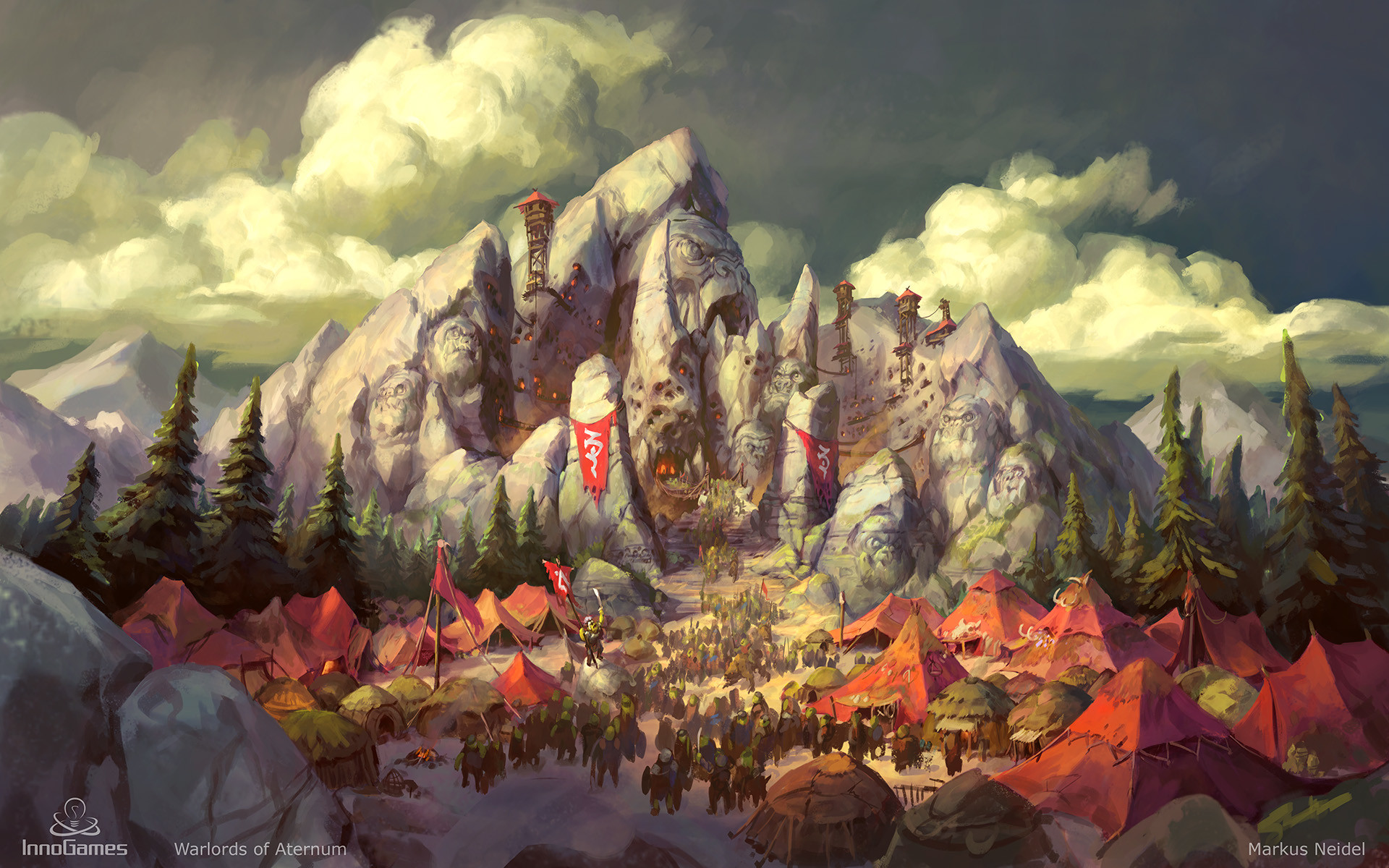This detailed painting by Marcus Neidell, titled "Warlords of Aeternum," showcases an ORC stronghold set against a dramatic backdrop of stormy gray skies interspersed with towering white cumulus clouds. The central focus is a jagged mountain peak, intricately carved with faces that range from menacing to slightly comical, evoking a sense of both magic and foreboding. The mountain's cliff sides are punctuated by watchtowers and red-roofed wooden cabins, connected by an intricate pulley system. Large red banners adorned with scrolling silver lines hang prominently from the rocky monoliths. 

At the base of the mountain, a dense forest of tall evergreen trees frames an extensive encampment. The camp is teeming with red canvas tents and grayish-green teepees, housing a mass of beings, possibly ORCs, dressed in heavy skins. These creatures appear to be moving between the camp and the mountain, possibly nearly a hundred in number. One figure stands on an elevated platform, arm raised, seemingly addressing the gathered assembly. In the foreground, gray boulders add depth and texture to the scene.

The painting features a soft, glowing light that illuminates the entire landscape, enhancing the fantasy ambiance. In the bottom left corner, the logo of InnoGames is visible alongside the game title "Warlords of Aeternum." The artist's signature, "Marcus Neidell," is in the bottom right corner, affirming the piece's origin and craftsmanship.